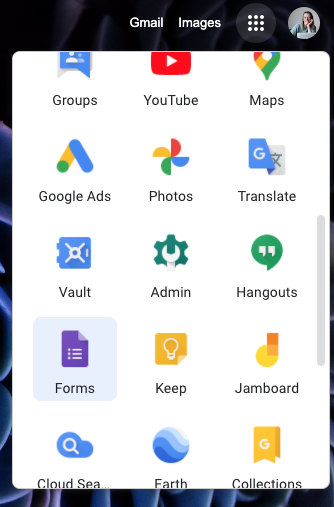The image shows the screen of a flat smartphone, likely a Google device, indicated by the predominance of Google-related apps. At the top of the screen, from the center to the right, there's a white status bar featuring various icons. These include signal strength, battery level, and a small square grid of dots symbolizing the app drawer. Additionally, there's a profile icon situated in the fifth row of the displayed apps.

The main area of the screen is a white background with several app icons arranged in a grid layout. The first row consists of icons for Groups, YouTube, and Maps. Following below, the second row includes Google Ads, Photos, and Translate. The third row showcases Vault, Admin, and Hangouts apps. The fourth row contains icons for Forms, Keep, and Jamboard. Lastly, the visible portion of the fifth row features Cloud, Docs, Earth, and Collections apps. Each app icon is distinct and most carry Google's signature color palette, reinforcing the likelihood that this is a Google smartphone. The presence of Gmail and other Google services further supports this conclusion.